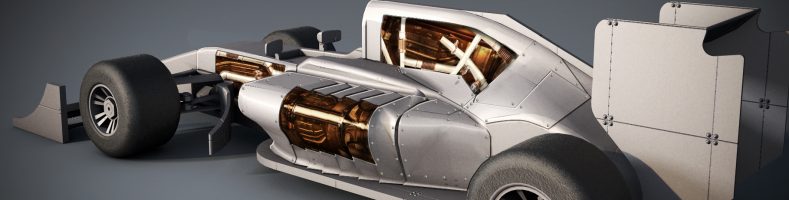This is a close-up 3D rendering of a sleek, silver model race car, reminiscent of those used in F1 or Grand Prix races. The image shows the car angled slightly from the right, with its aerodynamic form stretching from the front to the rear. The rear is partially cut off by the frame, revealing a boxy, silvery engine compartment that resembles a tail structure. The front of the car features a grey scoop, similar to a miniaturized bulldozer blade, leading into a slender, silvery grey center flanked by smooth, textured tires; one on the left fully visible, the other partially cut off on the bottom right.

Intriguingly, the car's silver exterior reveals glimpses of a brass interior with some exposed mechanical components, including a flanged cog and white dowels, visible on the side bump and in the driver's seat area. This area, possibly the cabin, is characterized by white tubes running across the brass interior. The vehicle is situated on a blue surface, enhancing the contrast with its metallic hues. Overall, the design melds textured and smooth surfaces, giving the race car a dynamic, high-tech look.